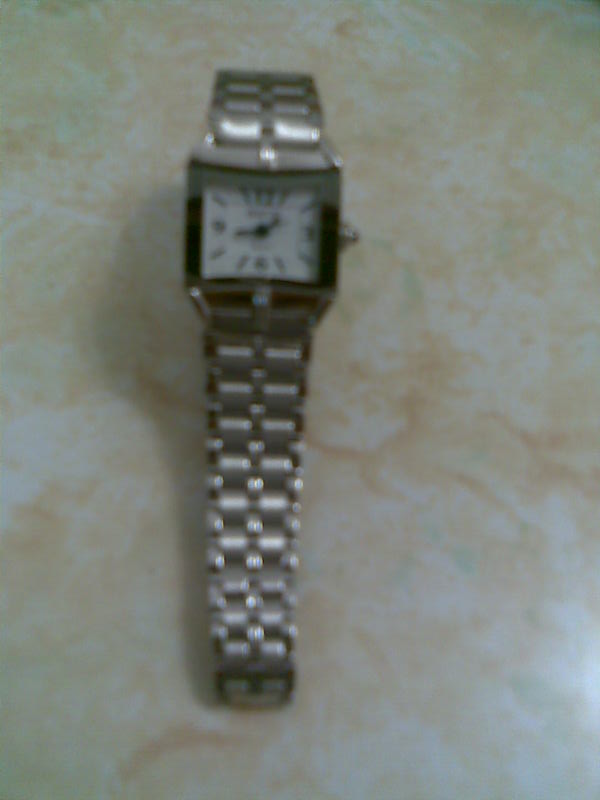A blurry photograph captures a wristwatch resting on a sleek, marbled surface. The table exhibits a striking marbled pattern with a white base interspersed with elegant brown striations. The wristwatch features a refined silver metal band and a distinctive rectangular face, suggesting it is likely a ladies' accessory. The watch face is white, adorned with bold black numerals at the 12, 3, 6, and 9 o’clock positions, while simple dashes mark the remaining hours. The time displayed is just past 8 o'clock, with black hour and minute hands providing clear contrast against the white background.